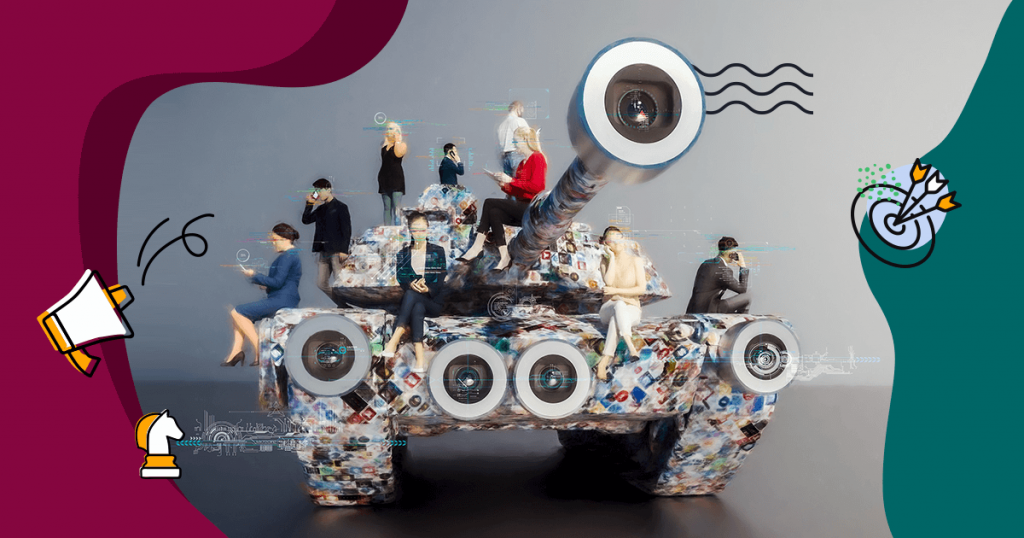The image features a horizontally aligned rectangular collage, predominantly shaded in hues of gray, with a dark red area on the left and a green area on the right. The left side includes a yellow and white megaphone icon and a chess knight piece in white and yellow. On the right, there are three black arrows, two with yellow backs and one with a white back, emerging from a black surface dotted with green.

The central object in the image resembles an army tank, seemingly constructed from various camera lenses and magazine cutouts, giving it a collage-like appearance. The tank's turret houses a camera lens in its cannon, with four additional camera lenses arrayed across the front of its body. Three horizontal, squiggly black lines extend from the top of the tank.

Surrounding the tank are several people, all engaged with their cell phones, either talking or looking at them. These individuals, dressed in business attire, appear in various positions: some sitting, others standing. Detailed descriptions of a few include a woman in a gray skirt suit, a man in gray pants and a blue or black shirt, a person in a blue suit, another in a red shirt and black pants, and a woman in all white. These figures contribute to the digitally manipulated and surreal atmosphere of the scene.

A white circle with blue outlines, positioned on the right, adds another layer to the strange, mixed-media effect of the composition. The tank itself stands on a surface shaded in darker gray tones, providing contrast to the lighter gray wall behind it. Overall, the image is a complex blend of military motifs, digital manipulation, and everyday human activity.